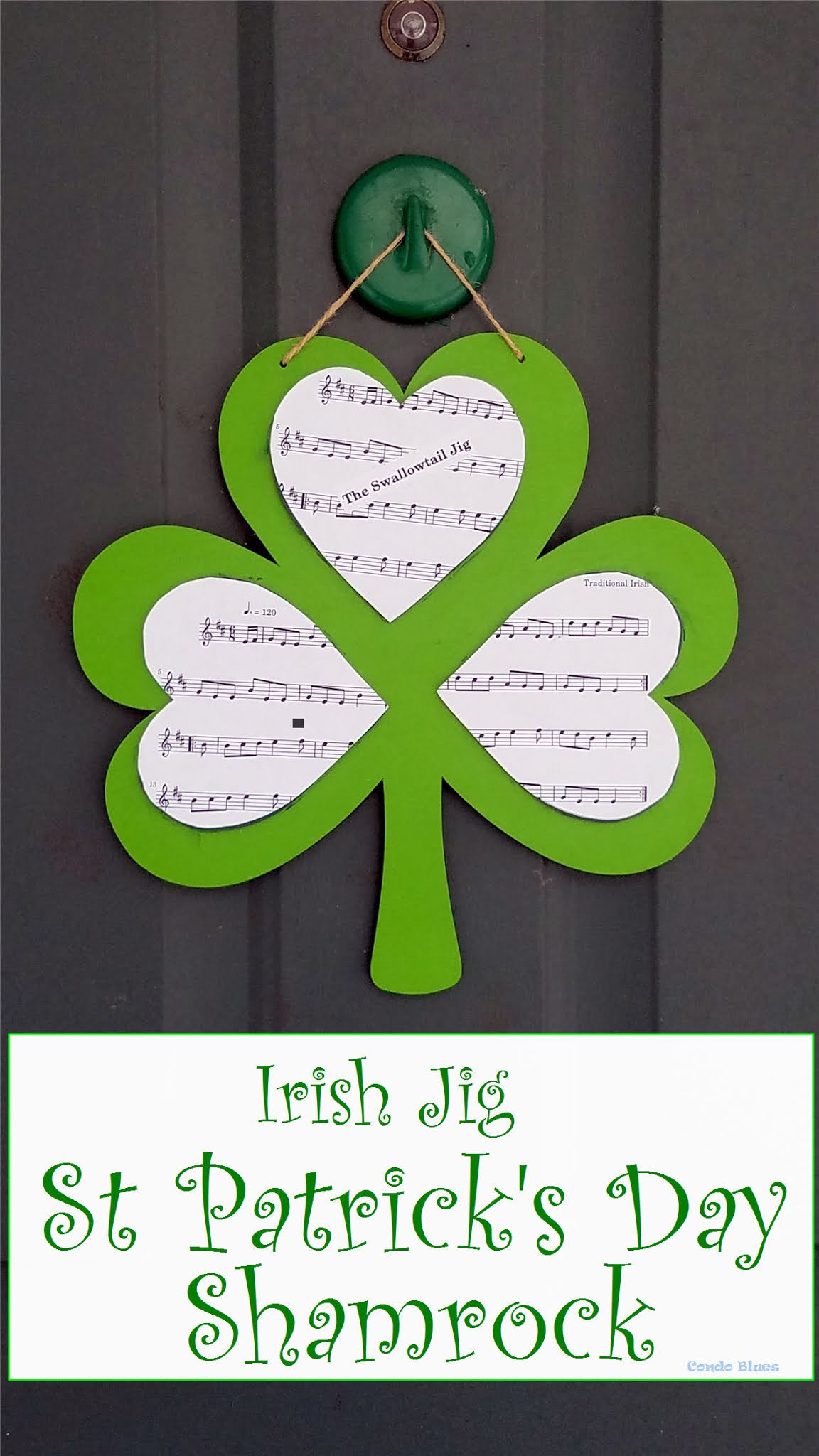In this detailed close-up photograph, a gray door features a prominent peephole at the top center. Beneath the peephole, a green hook securely holds an intricately designed paper shamrock. This charming decoration is crafted from green construction paper, forming a three-leaf clover. Each leaf of the clover has an additional layer—a heart-shaped cutout from sheet music, expertly displaying musical notes and titles. The top petal of the shamrock is labeled with "The Swallowtail Jig," and the leftmost petal includes tempo markings, making the sheet music notably detailed. Below this artistic arrangement, a digitally added banner with a whimsical, swirly green font on a white background reads "Irish Jig, St. Patrick's Day Shamrock." While this graphic element stands out from the paper texture of the shamrock, it complements the festive theme. The bottom right corner of the image contains an unreadable signature, suggesting a DIY or Pinterest-inspired creation.